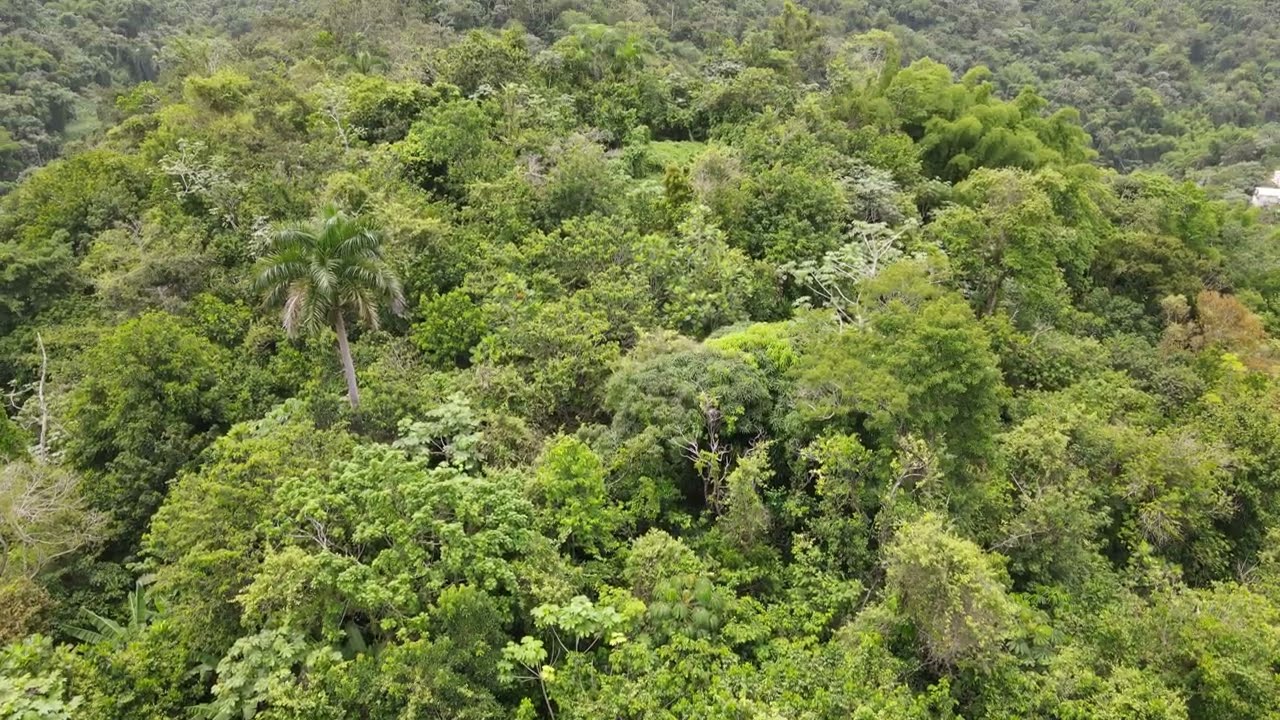This detailed aerial landscape photograph captures an expansive, densely packed forest or rainforest, shot from high above (likely from a drone or an airplane) in a horizontal orientation. The image showcases a vast grove of trees, predominantly characterized by their lush, green canopies. These round-topped trees form a continuous canopy with no visible skyline or horizon, emphasizing the sheer density of the vegetative cover.

A special point of interest is a tall, distinctive palm tree or tropical tree, located in the upper left-center of the image. This palm tree stands out remarkably, with its trunk extending several feet above the predominantly green, round canopies of the surrounding trees, drawing attention due to its height and different structure. The photo captures a variance in greenery, with trees displaying shades from very light to deep green, and even a few that appear dried up, almost brown.

The daylight filters through, casting a slight illumination on the treetops but avoiding heavy shadows, indicating the photograph was taken during daytime. Though predominantly capturing the natural beauty of the forest, the right-hand side of the image hints at human presence with what appears to be a couple of white houses, subtly blending into the dense foliage. Aside from these minor details, the photograph remains an undisturbed view of nature’s verdant expanse.